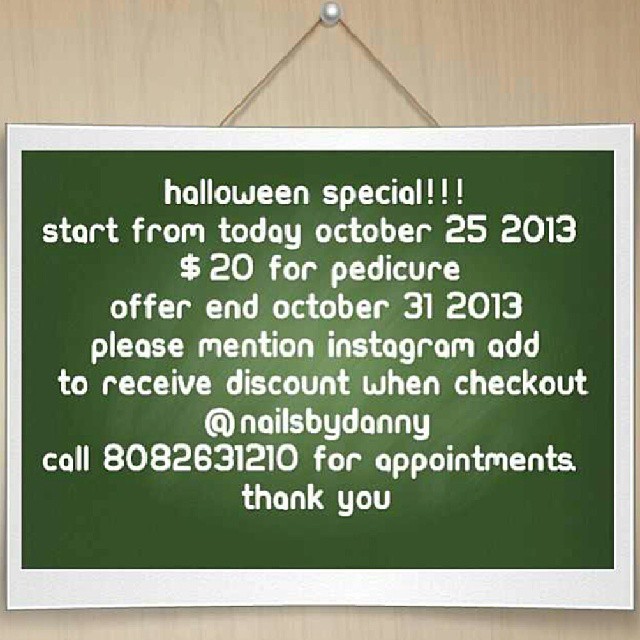A photograph captures a white sign prominently hanging on a wooden door, secured by a silver thumbtack. The sign features a Halloween special for Nails by Danni, with details presented in white letters on a central green square background. The advertisement announces a limited-time offer starting from October 25th, 2013, where customers can get a pedicure for $20. The promotion runs until October 31st, 2013, and requires mentioning an Instagram ad at checkout to avail of the discount. To make an appointment, potential clients are directed to call 808-263-1210. The sign's design, with clear and contrasting white text on a dark green background, is visually appealing and easy to read, ensuring that Danni's business gains visibility and interest during the Halloween season.